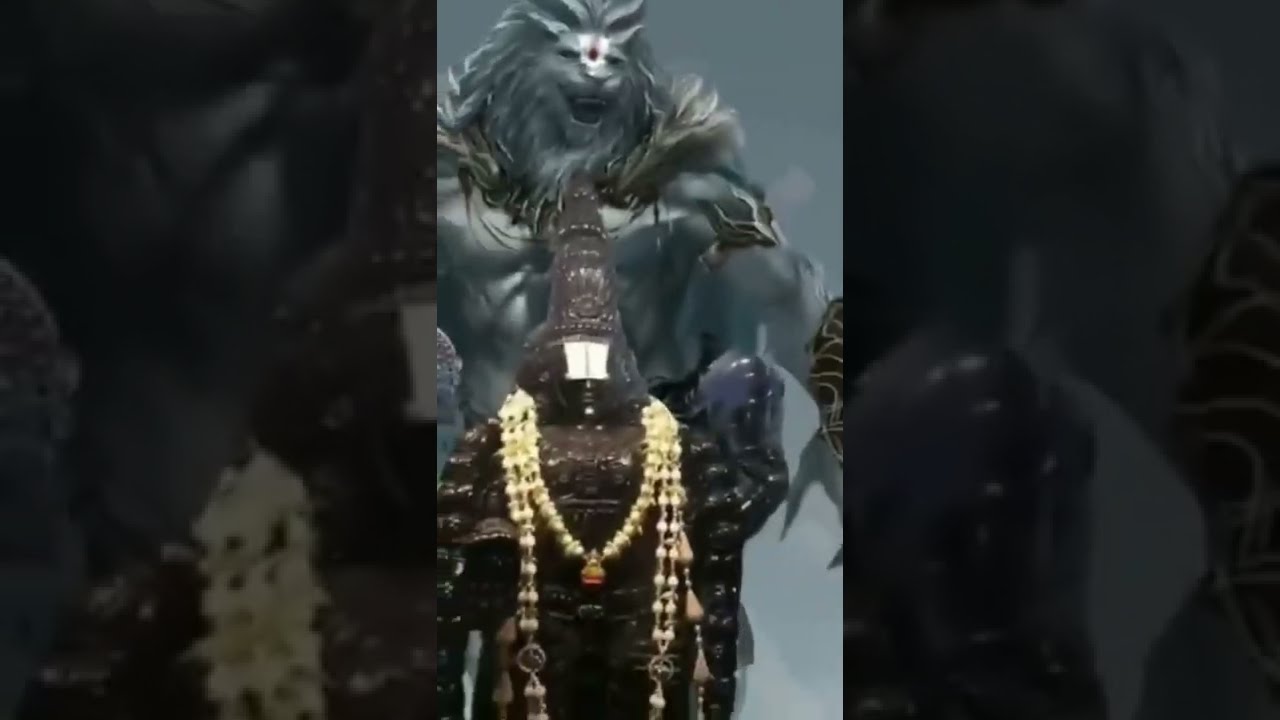The image shows a scene from a video game, featuring two fantasy creatures set against a dark, blurred background. Dominating the scene is a towering, anthropomorphic lion creature with a human-like chest and arms, adorned with armor. The lion creature's face, marked by a white war paint stripe running between piercing eyes down to its nose, is surrounded by a massive mane. Its mouth is open, revealing sharp teeth. The creature has long, sharp claws on its left hand, while the right hand is obscured by darkness. It wears a breastplate that extends into its pants, decorated with jewels hanging from a beaded necklace, and a lantern is attached to the center of the chestplate, just above the waist.

In front of the lion creature stands a smaller, heavily armored figure, draped in shiny brown armor and marked by a tall, pointy helmet with a white front. The figure's face is shrouded in dark brown, almost blending into the shadows. Golden chains adorn the armor, with one major chain hanging down the neck and additional chains draped on both sides. The lion creature's shoulders and wrists are also covered in armor, and a fur-like cloak cascades down its back. The overall image is presented in a portrait orientation, with the central focus bordered by an enlarged, fuzzier version that fills out the rectangular frame, adding to the dark, mysterious atmosphere. The background remains indistinct and gray, contributing to the image's ethereal quality.